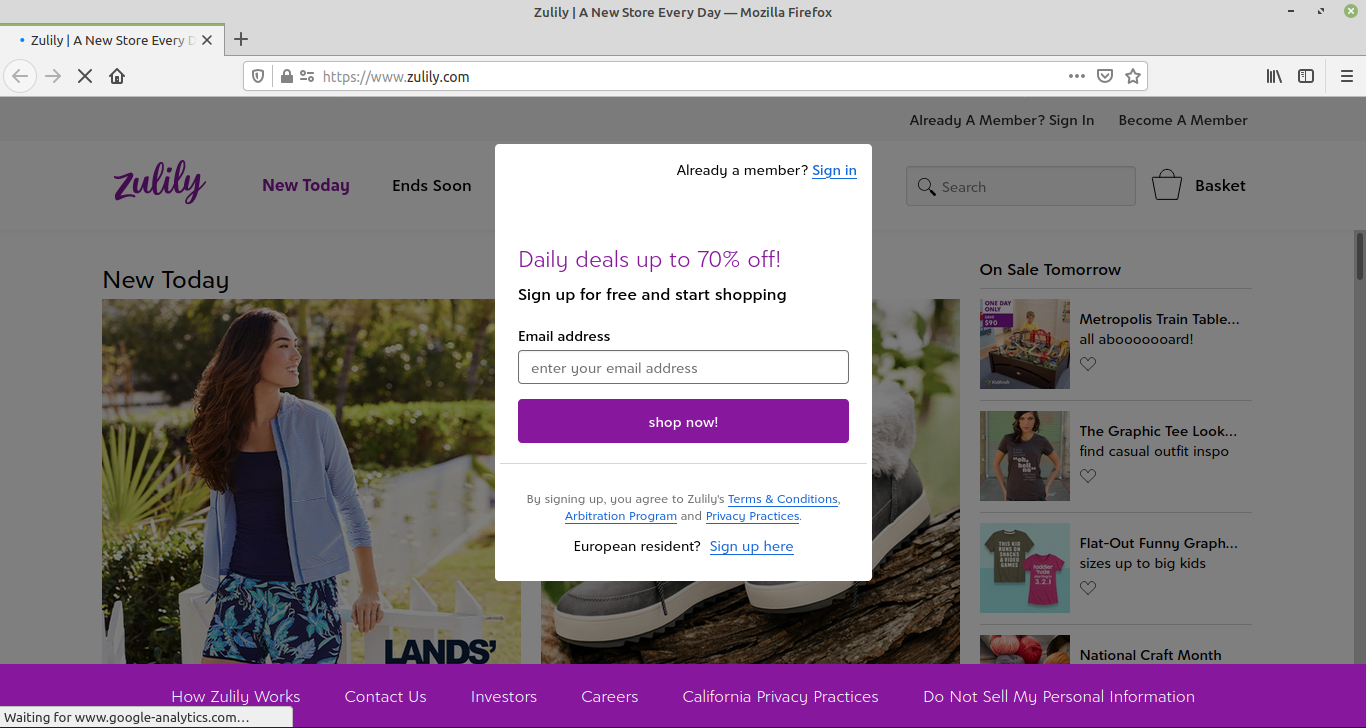In the screenshot of a Zulily website, a prominent white pop-up box is at the center, overlaying the muted main webpage. At the top of the pop-up, the text "Already a member? Sign in" stands out, with "Sign in" as a clickable hyperlink. Below, "Daily deals up to 70% off" is highlighted in striking purple to draw attention. The message "Sign up for free and start shopping" encourages new users, accompanied by a long rectangular box prompting users to "Enter your email address."

A large, eye-catching purple button reads "Shop Now," inviting immediate action. Further down, there's a note for European residents to "Sign up here," along with links to the "Terms and Conditions," "Arbitration Program," and "Privacy Practices."

The main webpage, although subdued due to the pop-up, showcases various elements. The top header features "New Today" in elegant purple text, and the word "Zulily" is written in a graceful cursive font. The brands available on the site include Land's End, and visually, there's an appealing image of a young girl modeling a stylish outfit: a cardigan over a black tank top and floral shorts, standing by a quaint white picket fence. Behind the pop-up, a display of shoes adds to the shopping allure.